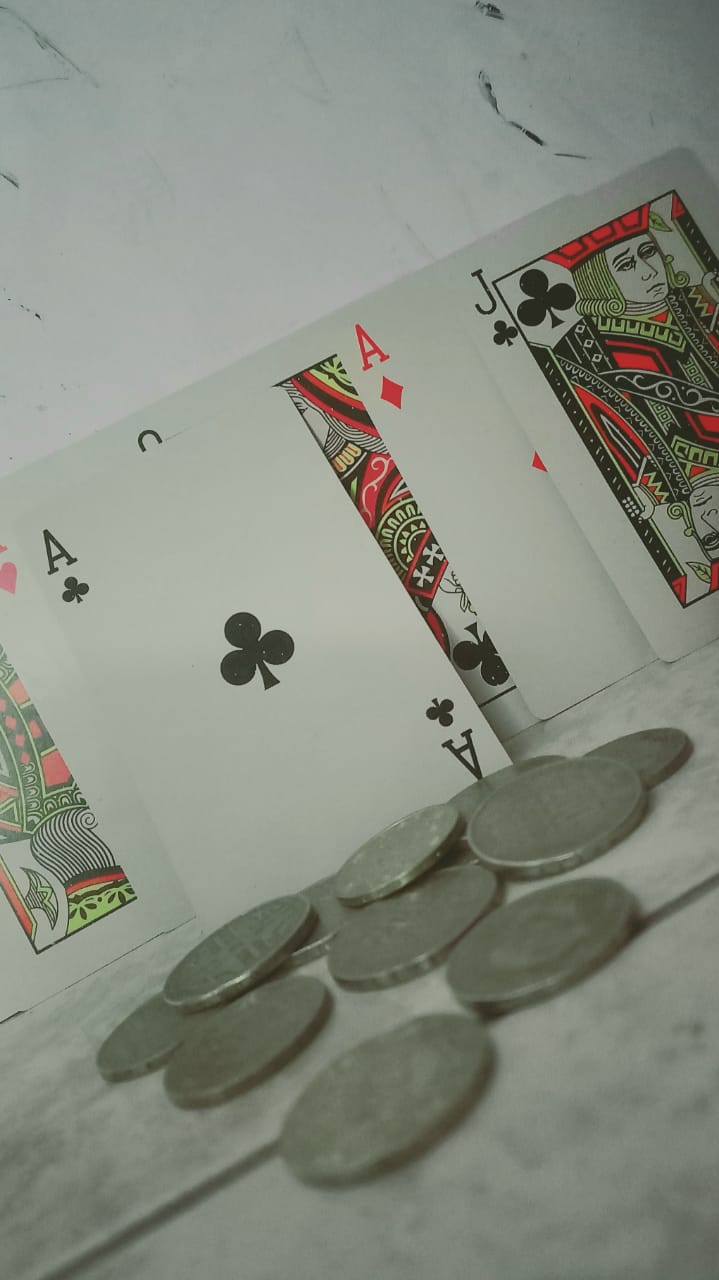In this photo, we see a collection of playing cards and coins arranged in an informal yet visually intriguing manner. In the background, six playing cards are stacked and slightly spread out, creating a line where each card overlaps the next without fanning out. The sequence of cards includes what appears to be a King of Diamonds, an almost completely obscured Ace of Hearts, an Ace of Clubs in the forefront, followed by a Queen of Clubs, an Ace of Diamonds, and a Jack of Clubs stacked horizontally. In the foreground, approximately ten coins are scattered haphazardly; though the fuzzy quality of the image makes it difficult to be certain, they seem to be nickels. The entire composition is set at a Dutch angle, tilting about 45 degrees to the left, adding a dynamic and unconventional perspective to the scene.